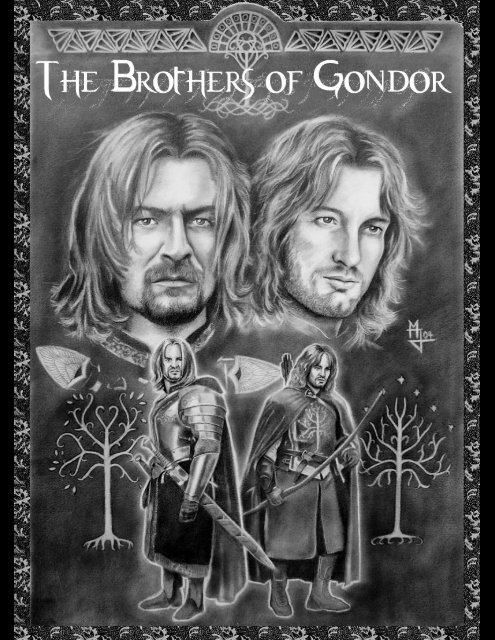This black-and-white image, possibly a book or DVD cover, features a detailed, textured border that resembles embossed leaves. A thin, solid black line frames the image, adding to its intricate design. At the top, on a smudged gray background, the title "The Brothers of Gondor" is prominently displayed in white capital letters. Below this are two illustrated fantasy characters with shoulder-length hair, beards, and mustaches. 

The man on the left, who appears older, has a thick mustache and a full beard, while the man on the right, who looks younger, sports a thinner mustache and a short beard with sideburns. Both men's facial expressions are composed, with closed mouths. Their illustrated heads appear close together, adding to the impression of brotherhood. 

Beneath these headshots, full-length images depict the men in medieval attire. The left figure is clad in full body armor, complete with a cape and a sword. The right figure, also in a cape, wears a chest plate and boots, and holds a bow. Flanking these characters are images of leafless trees, adding to the overall fantasy ambiance of the scene.